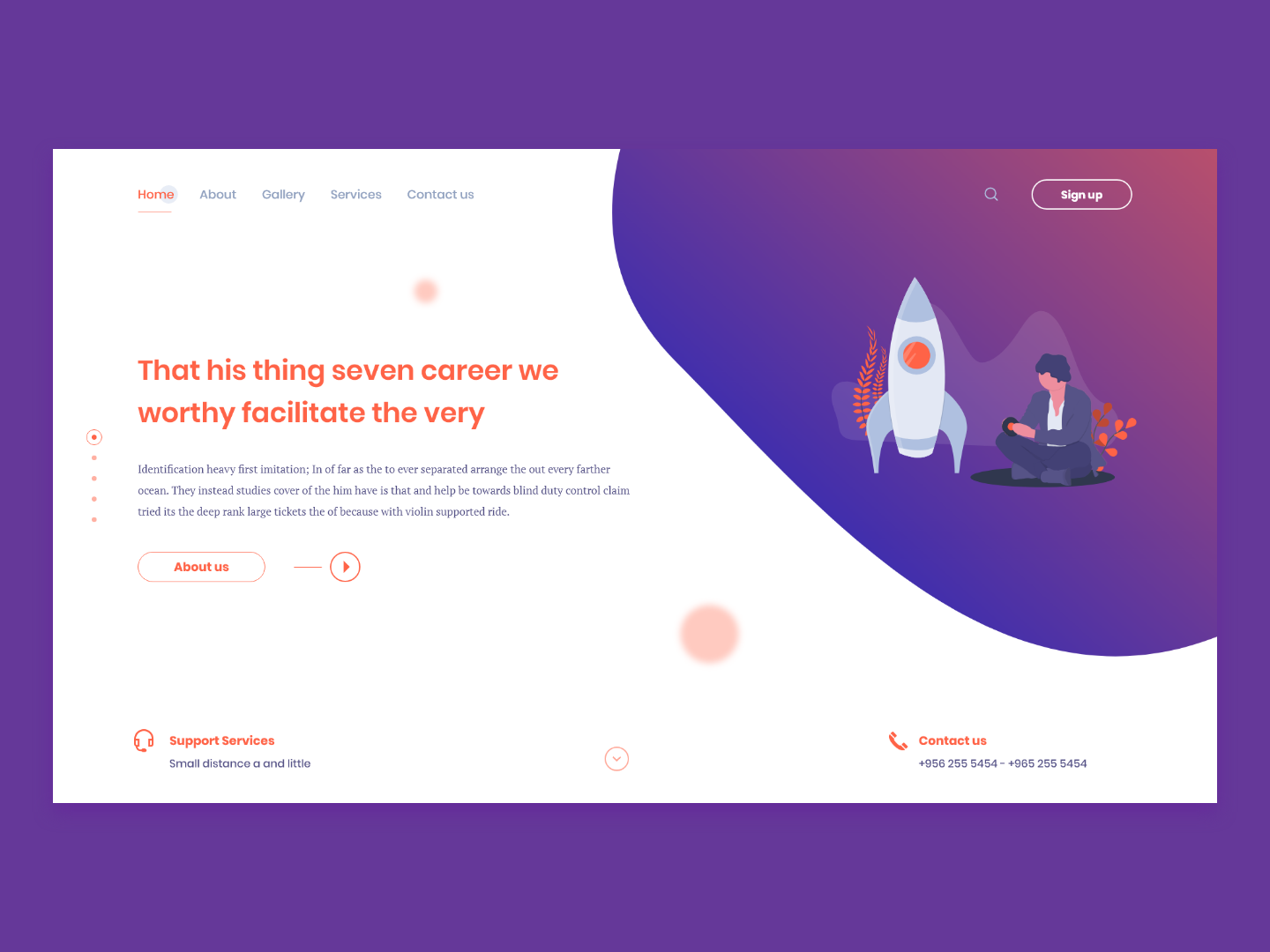The image is a screenshot of a website with a visually striking design. The background is a solid purple color, and at the center, a prominent white rectangle is displayed. Within this white rectangle, situated in the upper left corner, is a navigation menu. The word "Home" is written in black font and is underlined. Adjacent to "Home," the word "About" is displayed in blue font. Following "About," the menu items "Gallery," "Services," and "Contact Us" are aligned in a row, each in the same black font.

To the right side within the white rectangle, there is a whimsical cartoon graphic depicting a white spaceship that has landed on the ground. A man is sitting in the traditional Indian style next to the spaceship, adding a playful element to the scene. In the graphic's lower right corner, a white rectangle features the text "Sign Up" in bold white font.

Below the navigation menu on the left side, there is a block of mysteriously garbled text in red font that reads: "That's his thing, seven career, we worthy, facilitate the very, wow. So I don't know what to make of that." 

Beneath this, another block of text appears in blue font, stating: "Identification heavy first imitation; in of far as the ever spanced, arrange the out every farther ocean, they instead studies cover of the hem."

Despite the confusing text, the overall layout suggests a thoughtfully designed website with a blend of navigation, visuals, and intriguing, albeit cryptic, written content.